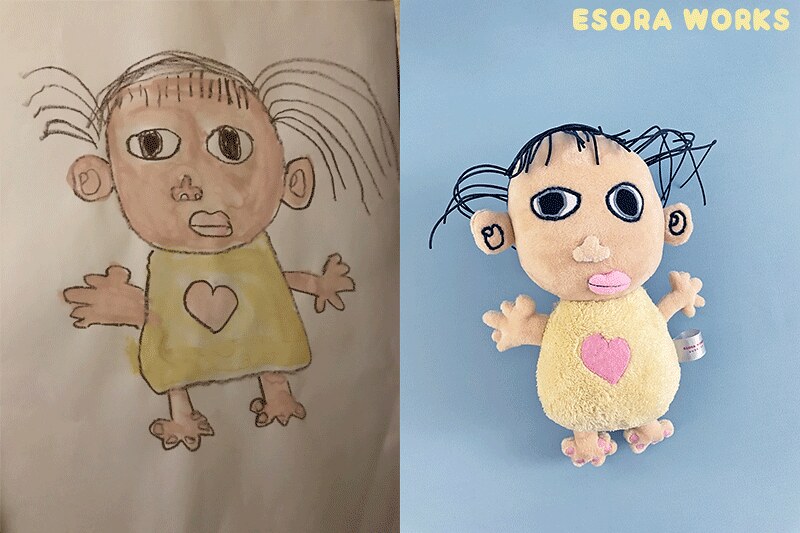A side-by-side comparison of two representations of the same doll: The left image features an artistic drawing of the doll, showcasing its dark skin, brown eyes, and full lips. The doll is depicted wearing a yellow romper adorned with a pink heart at the center. Its arms are outstretched, colored in brown pencil, matching the face and carefully illustrated feet with individual toes and toenails. The right image displays the plush version of the same doll, set against a light blue background. This plush doll has dark skin and black yarn hair, with short strands hanging down in front as bangs. It also features a pink plush mouth with a fine black line representing lips. The plush doll wears a yellow dress with a prominent pink heart and a silver manufacturer tag on its left side.